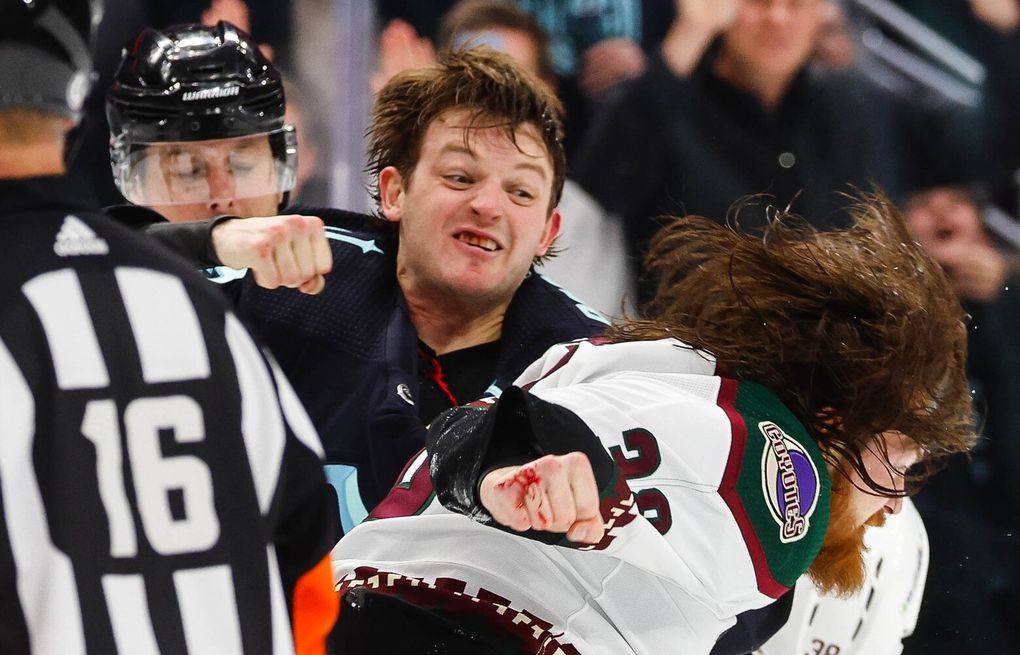The photograph captures a tense moment in a men's hockey game where a fist fight has broken out on the ice. Central to the image is a fierce confrontation: a player with bloody teeth, a furious expression, and clenched, bloody knuckles stands prepared to punch an opponent. This aggressive player, with fists raised, is marked by his intensity and visible anger. The man about to be punched is distinguishable by his long, flying hair, bushy red beard, and a Coyotes jersey, leaning forward with his eyes closed, seemingly bracing for the hit. Adjacent to the altercation is a referee in a black and white striped jersey with a red sleeve on his right arm, displaying the number 16, watching the scene unfold. Behind the chaotic scene, the audience is blurred but noticeably engrossed in the action, adding to the charged atmosphere of the photograph.